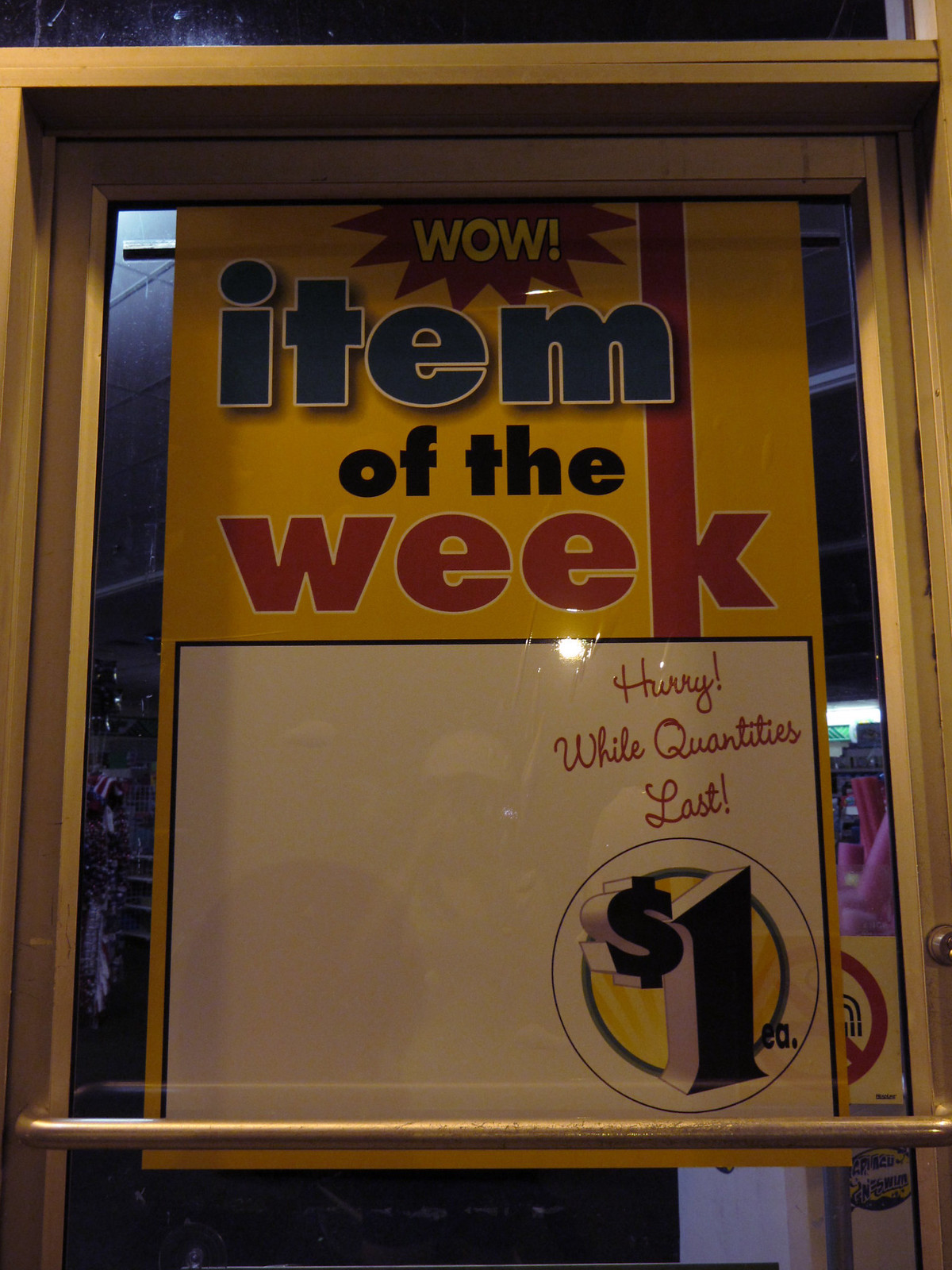In this vertically oriented, rectangular photograph, we are presented with an exterior view of a store window, framed in a brass color. The glass window is adorned with a vibrant yellow and white sign that immediately captures attention. Within the store, it seems to be closed, as indicated by the single, distant light visible in a back corner. The prominent sign on the window proudly declares "WOW, item of the week" in bold, block letters. Just below this proclamation, a smaller line of cursive text urges, "HURRY, while quantities last." Lastly, the most important detail—highlighted in black, block-lettered numbers encircled for emphasis—announces the price: "ONE DOLLAR EACH."